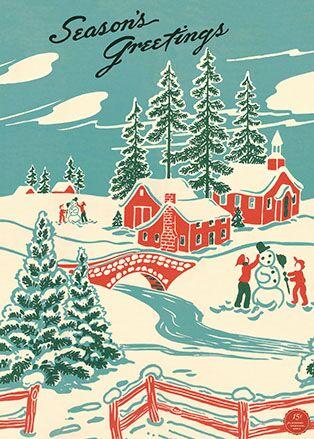This detailed holiday card features a nostalgic, vintage-style painting reminiscent of the 1920s or 1930s. At the top in elegant cursive text, it reads "Season's Greetings." The scene is set in a snow-covered winter landscape, with a vibrant blue sky filled with scattered white clouds overhead. 

In the foreground, a quaint red fence with an open gate stretches across the snowy ground. Dominating the scene is a charming red and white bridge crossing a bluish-green stream that meanders horizontally through the image. Majestic pine trees rise tall against the skyline, their evergreen branches contrasting sharply with the snow, and some children dressed in red and green winter clothes are constructing a snowman, with one child about to place a hat on its head.

The background of the card reveals more of the picturesque village. Several buildings, including a prominent red church and another large home, show their snow-capped rooftops. Beyond these structures, additional children can be glimpsed, busy with their own snowman creation amidst green trees dotting the snowy expanse. This idyllic winter scene captures the essence of a vintage Christmas celebration.